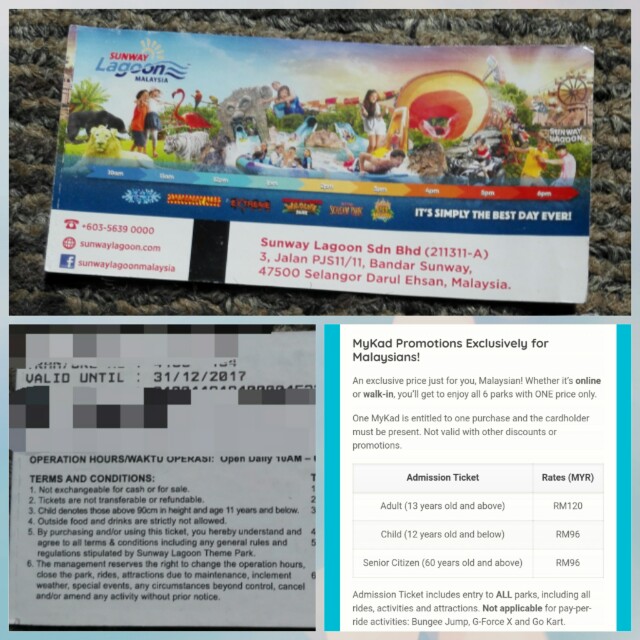Here is the cleaned-up and detailed caption for the image:

---

The image depicts a rectangular ticket stub set against a gray and black flecked granite countertop. The image itself is square, bordered predominantly in gray, with the left side transitioning to blue and extending about halfway across the bottom edge.

The ticket stub is vividly colorful, featuring an array of photographs including people, dogs, a Ferris wheel in the upper right corner, a child on a waterslide in the center, and flamingos, suggesting offerings like an amusement park and safari park. The ticket reads "Sunway Lagoon Malaysia," accompanied by various sponsor logos and the phrase "Simply the best day ever." The ticket is elongated in shape.

In the bottom left corner of the ticket, a white rectangle with red writing contains an old-fashioned telephone logo, a phone number, a tiny fleur-de-lis, a website name, and a Facebook logo with its corresponding address. Adjacent to this, a black or brown vertical bar resembles a magnetic stripe.

At the bottom right, a long white bar with red writing spans about two-thirds of the ticket's width. It reads, "Sunway Lagoon SDN BHD 3 Jalan," followed by a detailed address listing, "Bandar Sunway, 47500 Selangor Darul Ehsan, Malaysia."

The lower half of the image is divided into two squares. The left square, which is gray and white and pixelated at the top, contains the text "Valid until 31.12.2017," signifying an expiration date of December 31, 2017. Below this, a small font outlines "Operation hours, terms and conditions," followed by a six-item numbered list detailing these terms and conditions.

The right square, bordered by vertical turquoise bars, features the bold text "MyKad" with capitalized M and K, and announces a promotion exclusively for Malaysians. The text exclaims, "An exclusive price just for you, Malaysian!" and details that Malaysians can enjoy admission to all six parks with one ticket price, applicable both online and for walk-ins.